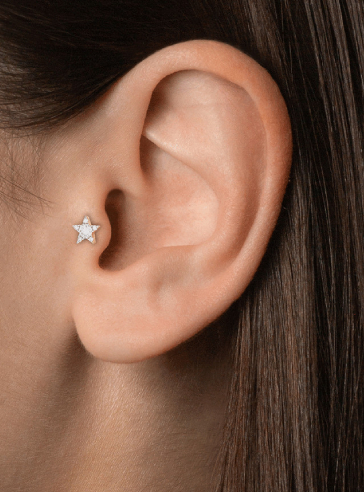This close-up photograph captures the left ear of a Caucasian female with fair, blemish-free skin and straight, thick brown hair. The hair is neatly tucked behind her ear, although a few stray strands and small, unshaved brown sideburns are visible. The focal point of the image is the tragus, adorned with a delicate diamond star stud earring. The photo also subtly reveals her ear canal, the natural contours and folds of her ear, her jawline, and a section of her neck. The lighting in the photograph is well-balanced, providing a natural and lifelike appearance with a good mix of contrast and vibrancy. The image likely serves as a professional product photo intended for a jewelry website.